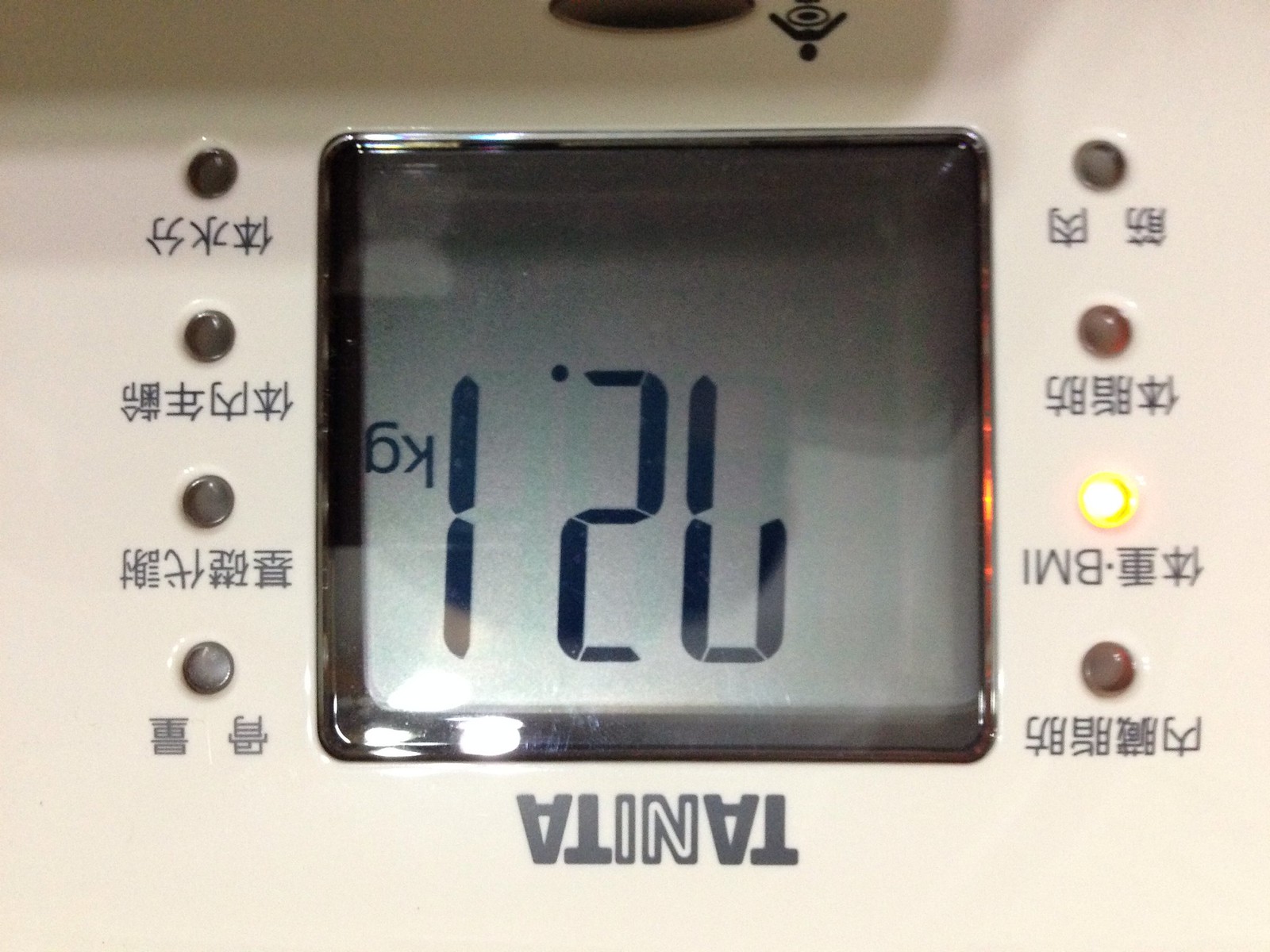The image depicts a close-up of a metal electronic scale, predominantly filling the frame without any visible background. The device is positioned upside down, revealing the brand name "TANITA" at the top. The letters "T-A-N-I-T-A" are stylishly presented with the "T-A"s in black and the "N-I" outlined in black but with white centers. An LCD screen displays the weight "72.1 KG" in dark blue characters. Surrounding the central display, there are four indicator lights on each side. The second light on the right, which reads "BMI" and is accompanied by Japanese text, is illuminated in orange. The other indicators are solely labeled in Japanese. At the top center of the scale, there is a symbol depicting a human figure with a highlighted circle around the stomach area, suggesting a focus on body measurements. The overall device has a light tan color, and the weighing area features a transparent glass panel.